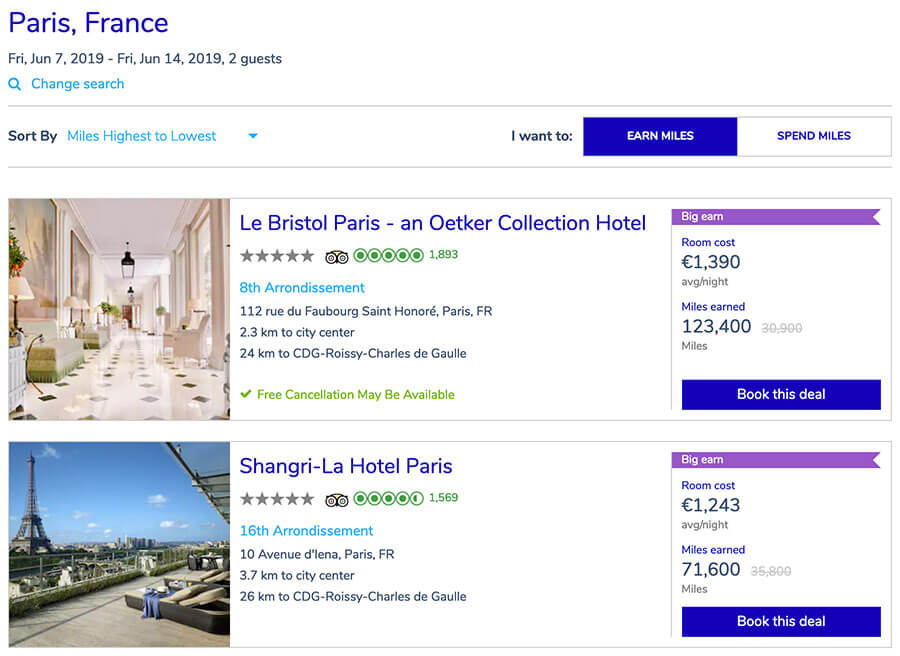**Caption:**

This image is a screenshot taken from a travel booking platform on a phone or computer, showcasing a selection of hotel listings for a trip to Paris, France. The interface has a clean, predominantly white background. At the top, the search parameters specify the travel dates as Friday, June 7th, 2019, to Friday, June 14th, 2019, for two guests. There's an option to "Change Search" beside a teal-colored magnifying glass icon.

Below these details, a sorting option reads "Sort by miles: Highest to Lowest." To the right, two buttons are displayed within a blue rectangle: "I want to earn miles" and "spend miles," with the latter option on a white background.

Further down, the listings feature high-end accommodations such as Le Bristol Paris and the Shangri-La Hotel. Le Bristol Paris is highlighted with a note indicating "Free cancellation may be available" in green text. The average nightly rate for this hotel is listed at £1,390. The Shangri-La Hotel in Paris is also displayed, with an average nightly rate of £1,243.